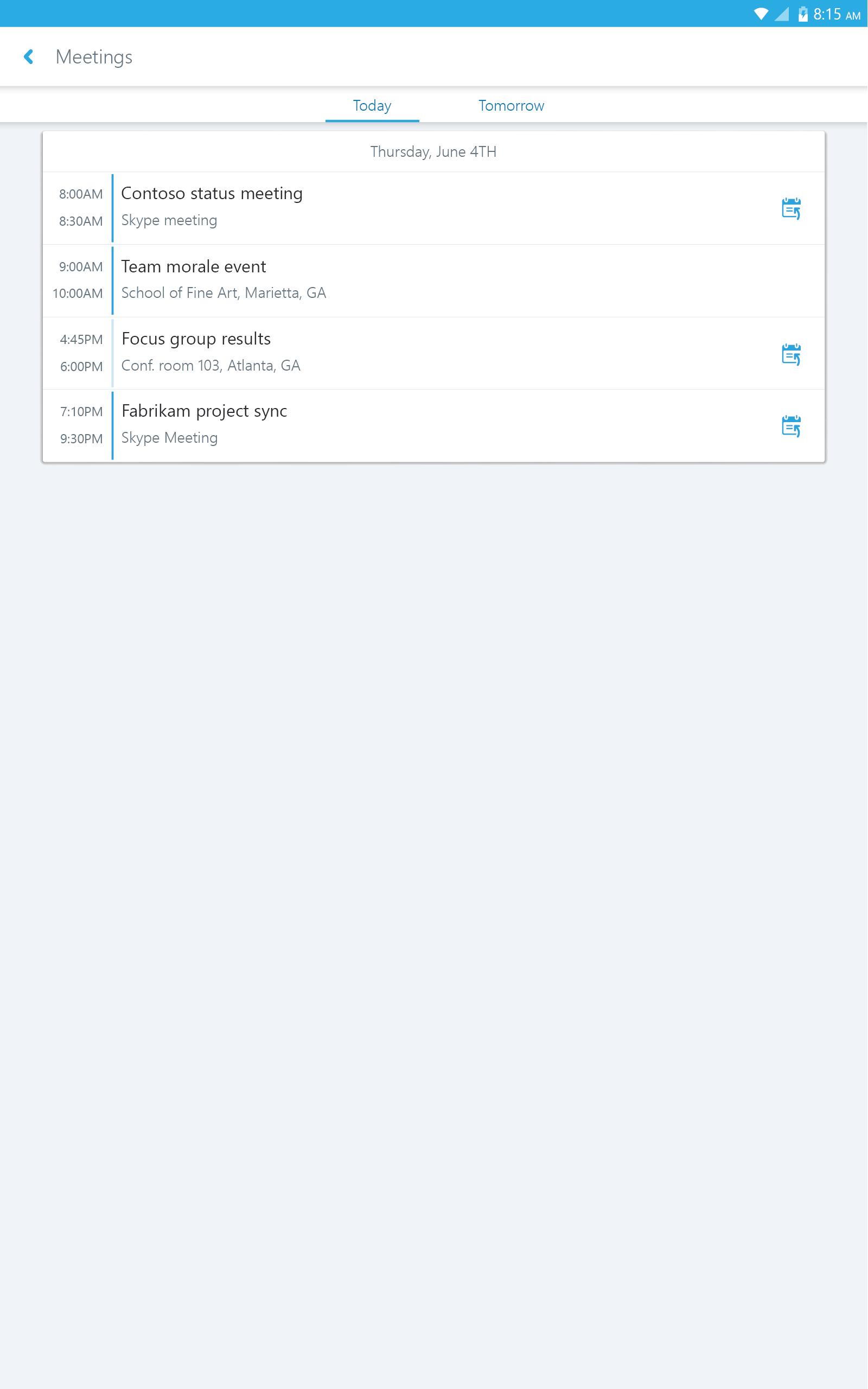This image is a screenshot of a computer screen displaying a detailed meeting schedule. The top portion of the screen features a light royal blue banner with the word "Meetings" prominently displayed. A blue arrow pointing to the left is also visible in this area. To the right side of the banner, there is essential status information including the current time, 8:15 a.m., and a battery life icon showing approximately 50% charge.

Underneath the blue banner, the screen is divided into a schedule view. At the top of this section, the word "Today" is underlined, indicating the current day's schedule, with "Thursday, June 4th" listed right below it. Adjacent to this, the word "Tomorrow" can be seen, suggesting an option to view the next day's meetings.

The left side of the schedule lists various meetings and events chronologically. The day's schedule begins at 8:00 a.m. with a "Contoso status meeting," followed by a "Skype meeting" at 8:30 a.m. At 9:00 a.m., there is a "Team morale event," and at 10:00 a.m., an event labeled "School of Fine Art Marietta, Georgia" is noted. Later in the day, at 4:45 p.m., there is a "Group results" meeting, and at 6:00 p.m., a session in "Conference room 103 Atlanta, Georgia." The schedule continues with additional entries, including a "Fabrikan project sync" and another "Skype meeting."

This comprehensive screenshot provides a clear and organized view of a busy day's agenda, reflecting a meticulous planning and scheduling effort.